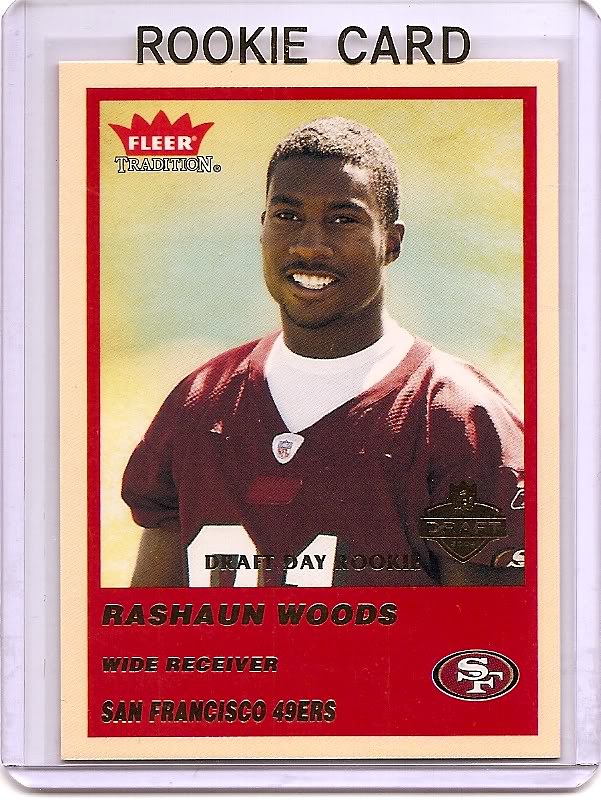This is an image of a collector's rookie card featuring football player Rashawn Woods. The card is securely wrapped in a plastic protective case. At the very top of the case, in black letters, it says "rookie card." The card itself is outlined with an orange border, coupled with a red line that encircles it. The background of the card is goldish. 

In the upper left corner, the card displays a crown-like emblem with the letters "FLEER" in white inside it, and beneath it, the word "TRADITION." Below this emblem is an image of the player, Rashawn Woods, who is an African-American man captured while smiling. He is dressed in a maroon or dark red football jersey with a white crew-neck shirt underneath. The jersey number is partially visible but not entirely clear. Behind him, there appears to be an open field. 

Near the bottom of the card, a black message reads "Draft Day Rookie." Further down, in a red box, it states "Rashawn Woods, Wide Receiver, San Francisco 49ers." Positioned at this red background's lower right corner, there is the San Francisco 49ers team logo.